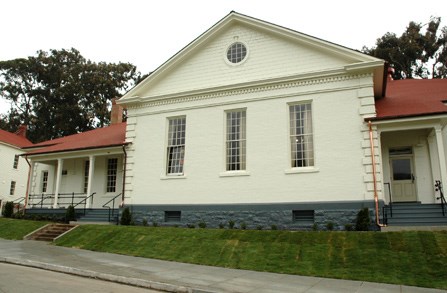This image captures a quaint, likely colonial-era house with distinct architectural features. The structure is painted a creamy white and has a striking red brick roof. The house, possibly used as a residence or business, features three long, narrow windows on the front and another set of three similar windows on the left side. At the forefront, a tan door with gray steps leads to the entrance, and there's another door and staircase on the left side. The house sits on a slight incline, necessitating stairs to reach the entrances. 

The foundation of the house is gray, matching the steps. Elaborate stonework on the eaves is adorned with small decorative balls that serve as a header, adding to the colonial charm. The property boasts a freshly mown green lawn on the incline, framed by tiny green bushes and flanked by two tall trees that provide some shade. In the foreground, a sidewalk and a hint of the street are visible, indicating a well-maintained and accessible property. The scene is set during the day, with the trees in the background completing the picturesque setting.